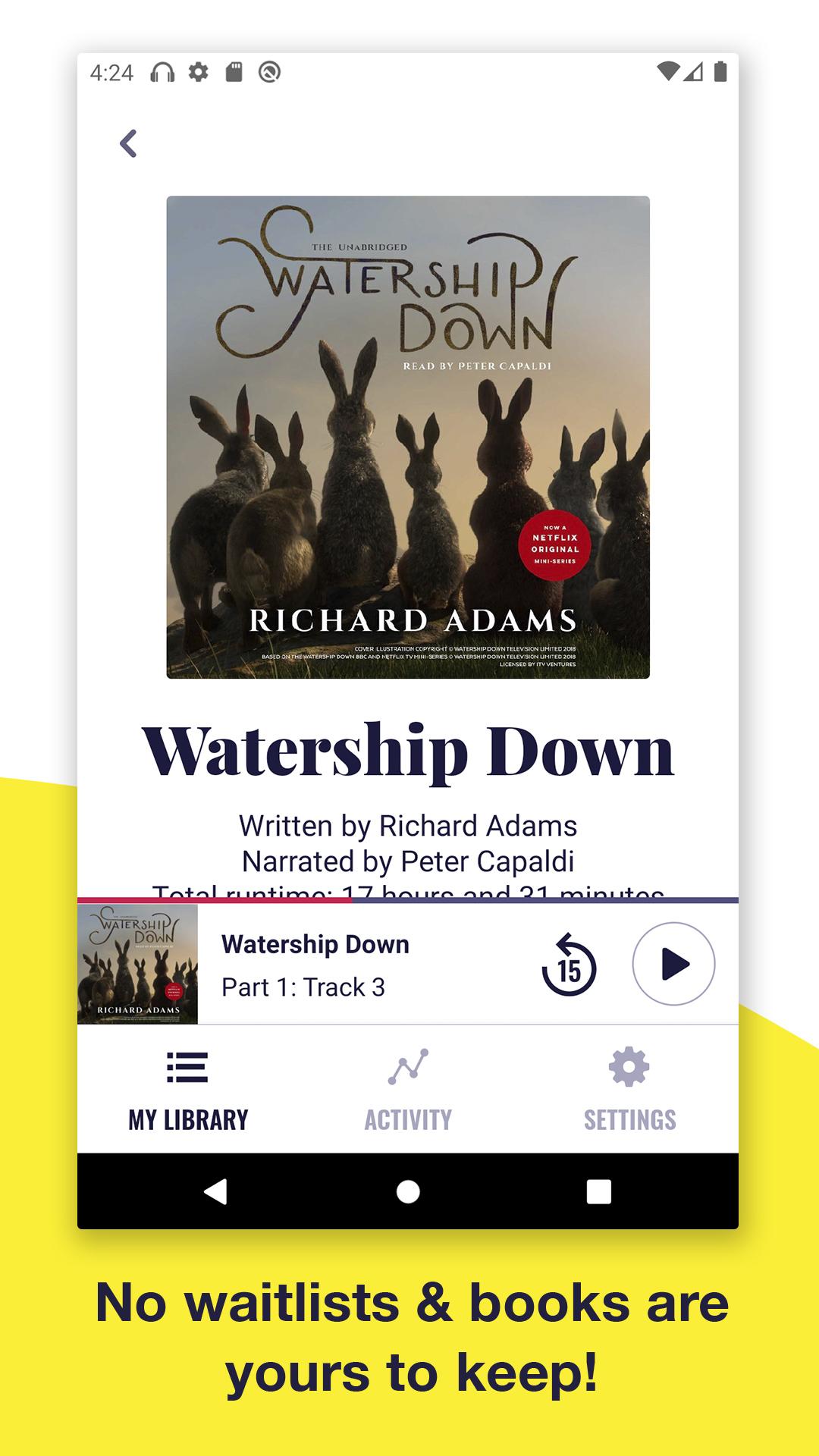In this vibrant advertisement for a music application on an Android cell phone, the focal point is a screenshot of the phone's screen. In the top left-hand corner, the time is displayed as 4:24. On the right-hand side, standard mobile indicators are visible, including a Wi-Fi signal icon, cellular signal strength bars, and a battery indicator.

Prominently displayed in the center is an album cover. The cover art features seven rabbits gazing off into the distant sky, setting a whimsical and imaginative tone. This album cover represents the music playing on the app, identified as "Watership Down" by Richard Adams.

Directly underneath the album art, the current song playing is specified: "Watership Down, Part One, Track Three." At the bottom of the screen, a caption reads, "No wait list and books are yours to keep," suggesting additional features of the application, such as possibly combining music with audiobooks or e-books without any borrowing queues. The overall image effectively highlights the user interface of the music app while also hinting at other versatile functionalities.